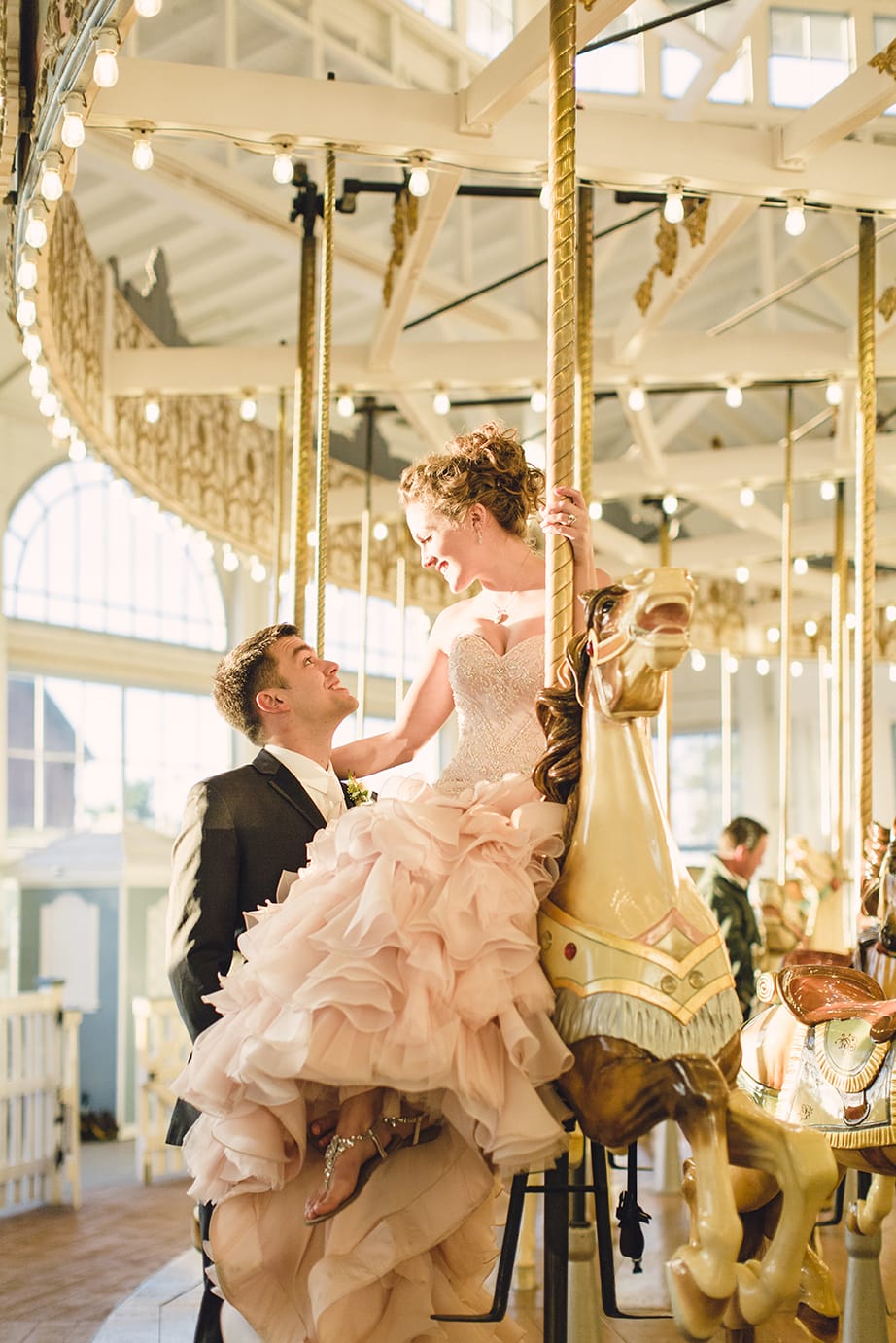The image depicts an elegantly staged engagement or wedding photograph of a white couple at a vintage merry-go-round adorned in gold and brown hues. The bride, a white woman with auburn hair, sits gracefully on a golden-brown wooden horse frozen in mid-run. She is adorned in a beautiful pink and white ruffled dress that flows with intricate furrows at the bottom, paired with flat, elegant shoes. The bride clings lightly to the golden pole, gazing affectionately at her groom below. Her groom, a white man with short, dark brown hair, dons a classic black and white tuxedo accentuated by a flower on his lapel. He stands on the carousel, looking up at her with love. The background reveals a white-themed entrance to the merry-go-round, with subtle decorative lights adding daytime ambiance, and another man can be faintly seen, possibly part of the fair or circus setting.